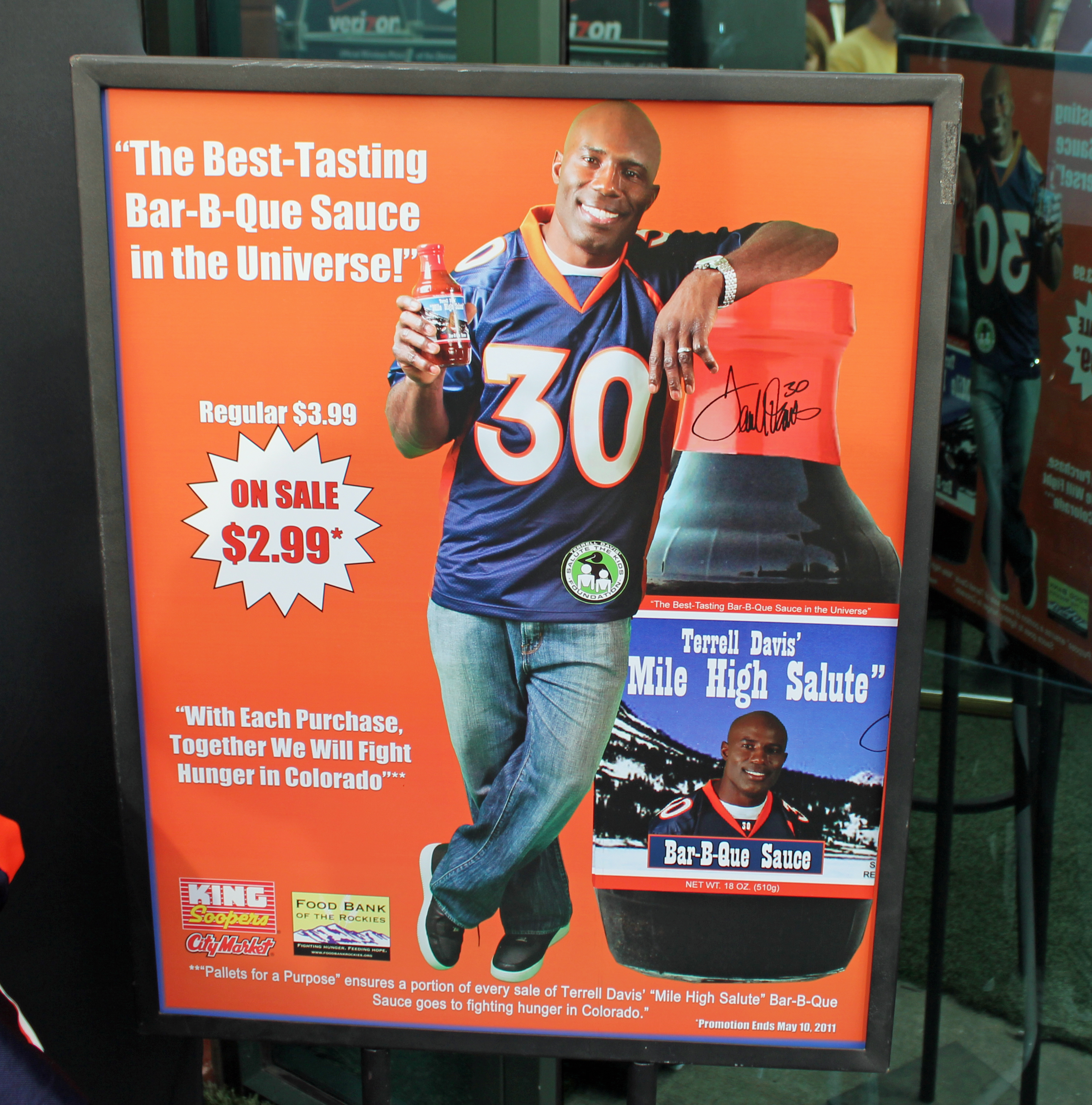The image is a color photograph of a freestanding, color-printed poster framed in black, set against an outdoor background. The poster prominently features professional football player Terrell Davis, a middle-aged, bald black man, wearing a blue football jersey with orange trim around the collar and the number 30 in white letters. He is also dressed in blue jeans and black and white sneakers. Terrell Davis stands in the center, fully visible from head to toe, holding a bottle of barbecue sauce in his right hand while leaning his left arm on a large, oversized bottle of barbecue sauce. The oversized bottle displays the text "Terrell Davis's Mile-High Salute Barbecue Sauce" towards the bottom right. The background of the poster is vibrant orange with white text. In the top left corner, the text reads "The best tasting barbecue sauce in the universe!" Below that, it advertises the price with "Regular $3.99" and "On sale $2.99" in a white burst with red type. Further down, it states, "With each purchase, together we will fight hunger in Colorado." The image style is photographic realism, capturing a promotional advertisement for Terrell Davis's signature barbecue sauce.